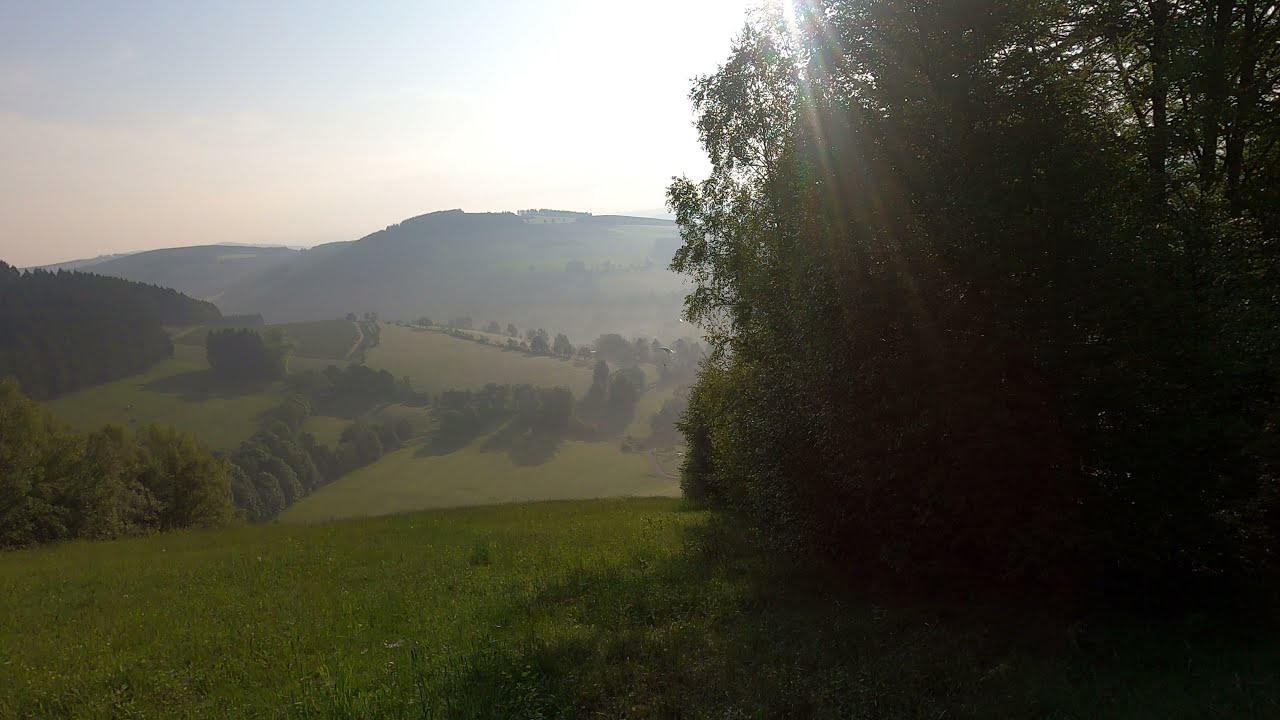The image captures a picturesque hilly countryside dotted with lush, short green grass, and bordered by dark green trees and hedges. A striking feature of the composition is the man in a parachute paragliding in the center, adding a dynamic element to the serene landscape. On the right side, thin trees cast long shadows, creating a contrasting interplay of light and shadow. In the distance, on a far hill stands a solitary white rectangular building with a flat roof, almost hidden by surrounding trees. The sky above varies from a light blue to a slightly hazy or smoky pinkish hue, cut by soft white clouds. The sun is visible at the top center of the image, its rays peeking through the leaves on the right, suggesting the time is around midday. There are no other buildings, animals, or people visible, making the rolling hills and well-kept pastures appear expansive and tranquil.